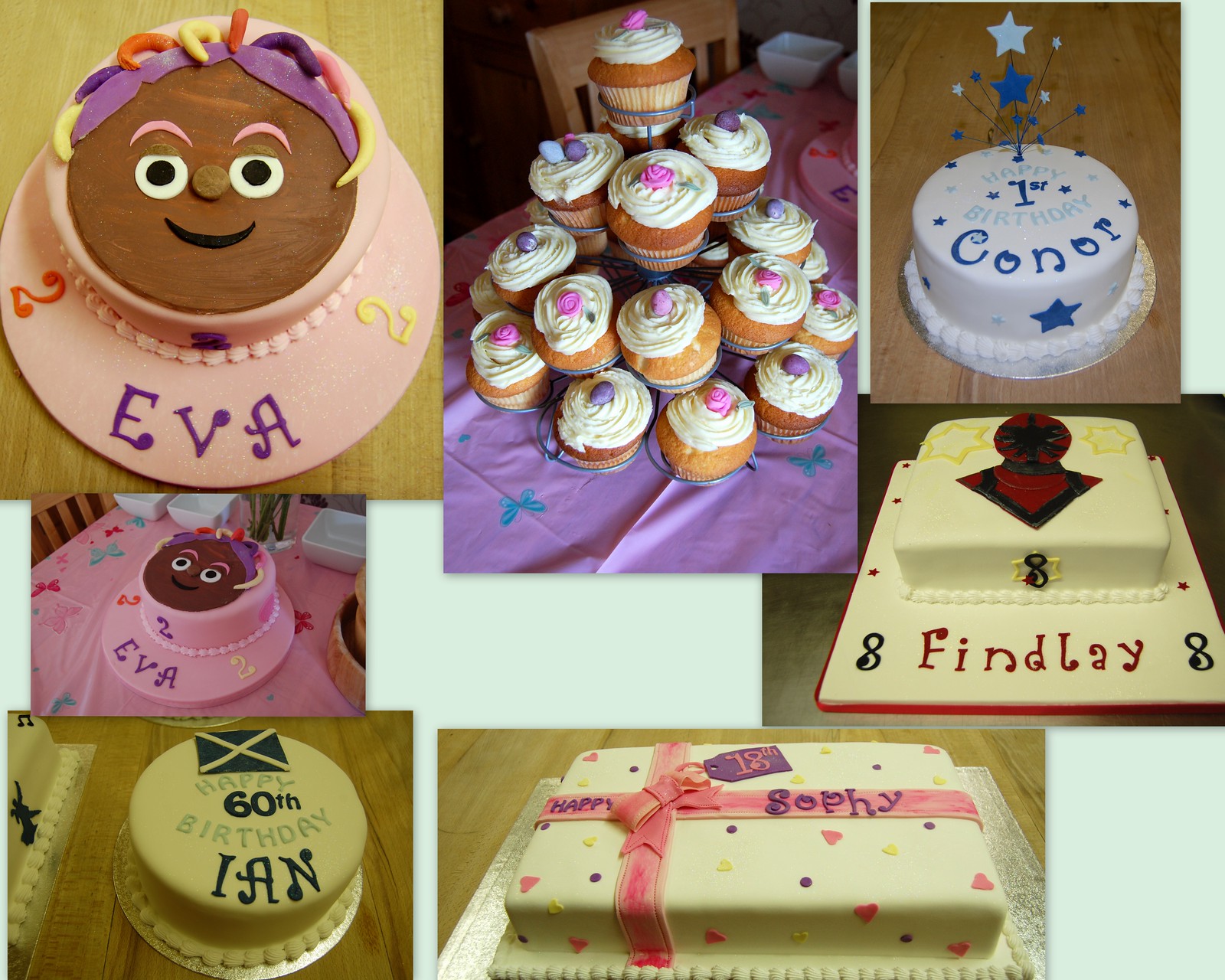This colour photograph is a detailed collage of various decorated cakes and desserts. In the upper left-hand corner, there is a round, fondant-covered cake designed to resemble a smiling face with purple and red "hair" and the inscription "Eva 2." Next to it, on the right, is a white cake decorated for a first birthday, featuring a blue star and the text "First Birthday Connor" in blue icing. To its left is an image of vanilla cupcakes, numbering around a dozen, all topped with white frosting and small pink or purple dollops. Further down on the left side, partially overlapping the face cake, is a pink cake also labeled "Eva 2," showcasing a similar design. In the upper right section, a square white cake features a Spider-Man motif and the label "8 Finley," written in red and black icing. Below this Spider-Man cake, occupying the central right part of the collage, is a Scottish flag-themed round cake with the message "Happy 6th Birthday Ian" in black icing. Finally, at the bottom right, a rectangular white cake is designed to appear like a wrapped gift, complete with a fondant pink ribbon, multicoloured hearts, and dots. The text "Happy 18th Sophie" is prominently displayed, with "18th" on a purple tag attached to the bow and "Happy" and "Sophie" written along the ribbon in purple icing. The photographs are slightly overlapping each other and are set against a cream-coloured background.